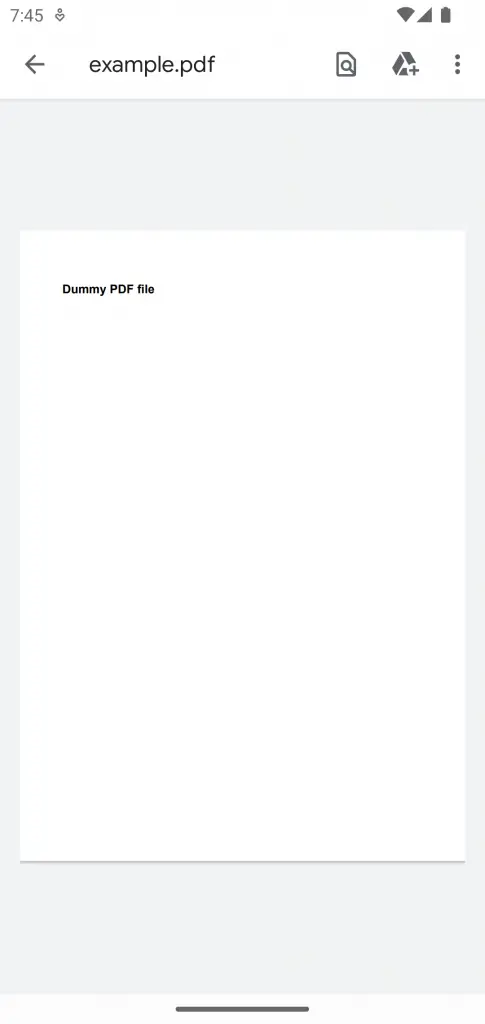**Detailed Caption:**

In this image, we see the interface of a PDF application displayed on an iPhone. The distinct characteristics of an iPhone are evident, including the prominent home bar at the bottom of the screen and the typical iOS heads-up display at the top. The interface primarily features white as the dominant color. The time is indicated as 7:45 in black text against a white background along the top of the screen. Additionally, an icon indicates that the microphone is active. 

On the right side of the top bar, there are three icons displayed in sequence, representing full Wi-Fi connectivity, full cellular reception, and a fully charged battery. Below this, the application bar displays the file's name, "example.pdf," with a back arrow on the left for navigation. On the right side of this bar, there's a "search in document" button depicted with a paper icon and a magnifying glass, a "save to Google Drive" button marked by the Google Drive icon with a plus sign, and a menu button represented by three vertical dots for additional options.

The main area of the screen has an off-white background with a white, portrait-oriented square in the center where the PDF content is displayed. Inside this white square, in the upper left corner, is the text "dummy PDF file" written in black. The rest of the page below this text remains empty, filled with white space, indicating a sample or placeholder document.